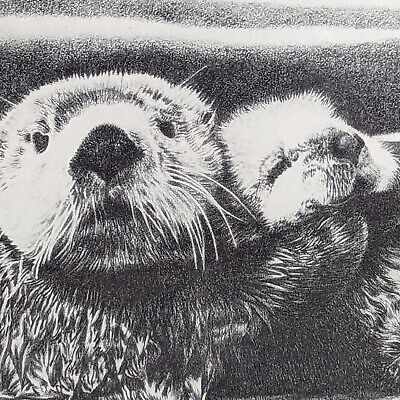The image appears to be a highly detailed pencil or pen-and-ink drawing, rendered in black and white, with all elements depicted in various shades of gray. It features a very close-up view of what seems to be a mother otter cradling her baby. The mother otter, positioned prominently in the image and taking up the majority of the frame, looks directly at the viewer with a slightly surprised or alarmed expression. Her large whiskers are clearly visible, and her paws are wrapped protectively around the baby otter to her left. The baby otter's eyes are closed, giving it a serene appearance. The background is blurred out, composed of a mix of black, gray, and white, providing no additional context. The overall impression is of an intimate and tender moment, despite the mother's seemingly concerned gaze.